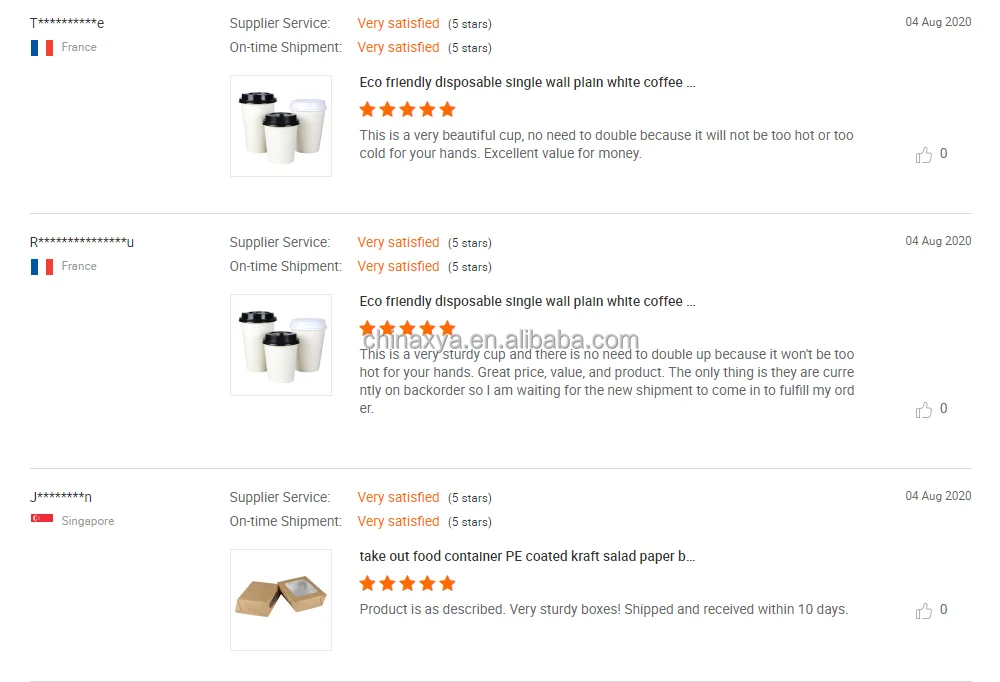Detailed Caption:

In the upper left corner of the image, there's a stylized logo featuring a capital "T" followed by a series of stars, and an "E" at the end. Below this logo is the vertically oriented flag of France with its tricolor bands of red, white, and blue, accompanied by the word "France."

On the right side of the image, several captions are displayed. They read: "Supply service: very satisfied," in orange for the heading, and below it, "Supply on-time shipment: very satisfied," in black. Additionally, the date "04-2022" is present in the upper right corner of all descriptions.

The first two items feature eco-friendly disposable plain white coffee cups, depicted as a set of three cups; two with black lids, and one with a white lid. The first coffee cup description highlights its aesthetic appeal and practical design, stating: "A very beautiful cup. No need to double as it will not be too hot or too cold for your hands. Excellent value." The second coffee cup review emphasizes its robustness: "A very sturdy cup. No need to double it as it will maintain a comfortable temperature for your hands. Great price, value, and product. Note: Currently on backorder; awaiting new shipment to fulfill the order."

The final item describes take-out food containers made of PE-coated Kraft shower paper. The containers are shown as small tan boxes with the accompanying text: "Very sturdy boxes. Product shipped and received within 10 days."

These detailed descriptions provide a comprehensive view of the products showcased in the image, highlighting their quality, design, and satisfaction ratings.